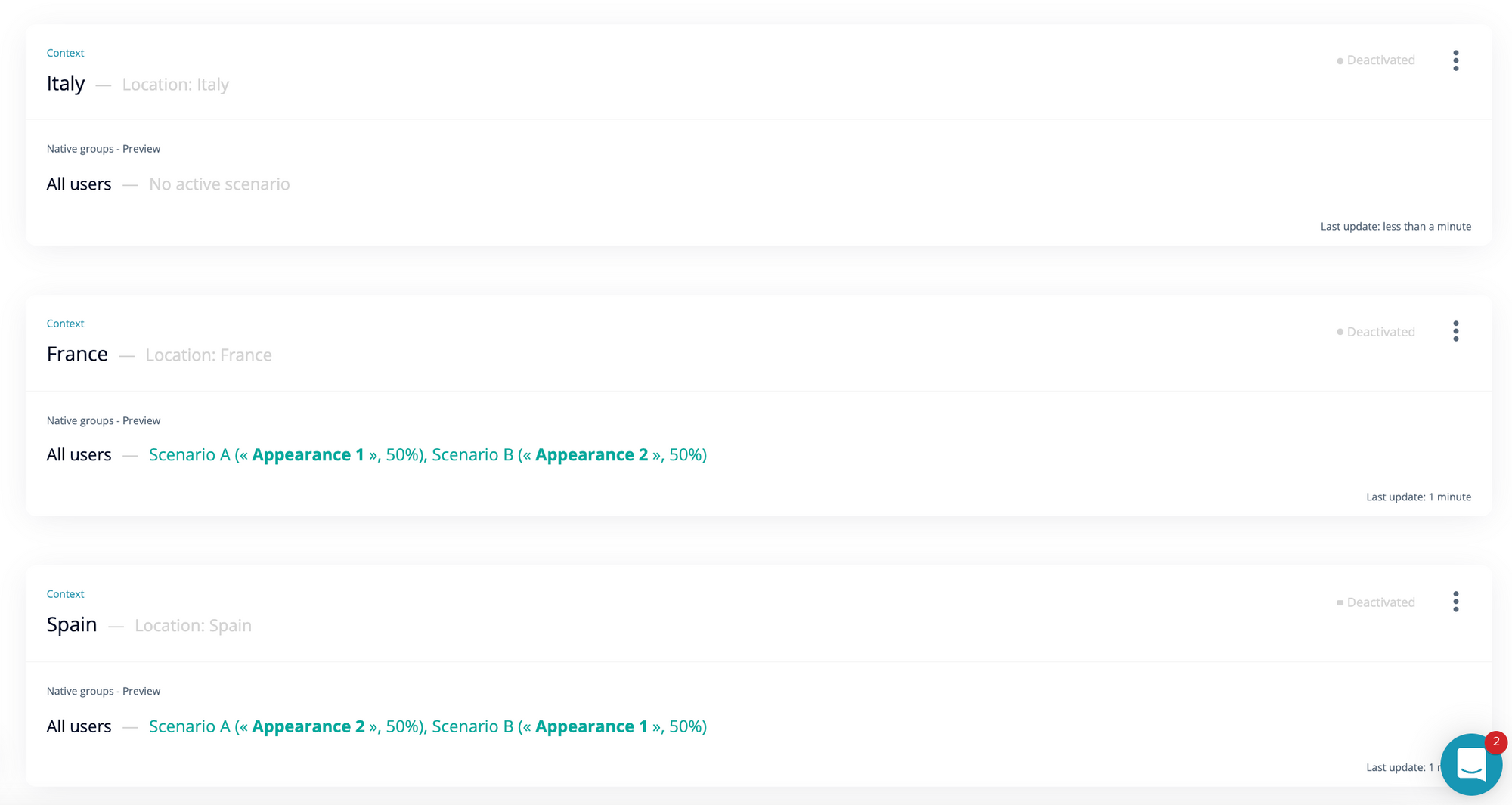The image consists of three horizontally arranged, white rectangular boxes, aligned vertically. 

1. **First Box (Italy)**:
    - Top left: "context" in tiny blue letters.
    - Below "context": "Italy" in black letters.
    - Next to "Italy": "location: Italy" in gray letters.
    - Far right: "deactivated" in gray letters.
    - Below this section: "native groups - preview" in gray letters.
    - Further below: "all users" in black letters, and next to it in gray, "no active scenario."

2. **Second Box (France)**:
    - Top left: "context" in tiny blue letters.
    - Below "context": "France" in black letters.
    - Next to "France": "location: France" in gray letters.
    - Far right: "deactivated" in gray letters.
    - Below this section: "native groups - preview" in gray letters.
    - Further below: "all users" in black letters.
    - Below "all users": "scenario A (appearance one 50%) scenario B (appearance two 50%)" in blue letters.

3. **Third Box (Spain)**:
    - Top left: "context" in tiny blue letters.
    - Below "context": "Spain" in black letters.
    - Next to "Spain": "location: Spain" in gray letters.
    - Below this section: "native groups - preview" in gray letters.
    - Further below: "all users" in black letters.
    - Below "all users": "scenario A (appearance two 50%) scenario B (appearance one 50%)" in blue letters.
    
In the bottom right corner of the image, there is a text message icon. The icon is white and situated within a blue circle, indicating two unseen notifications.